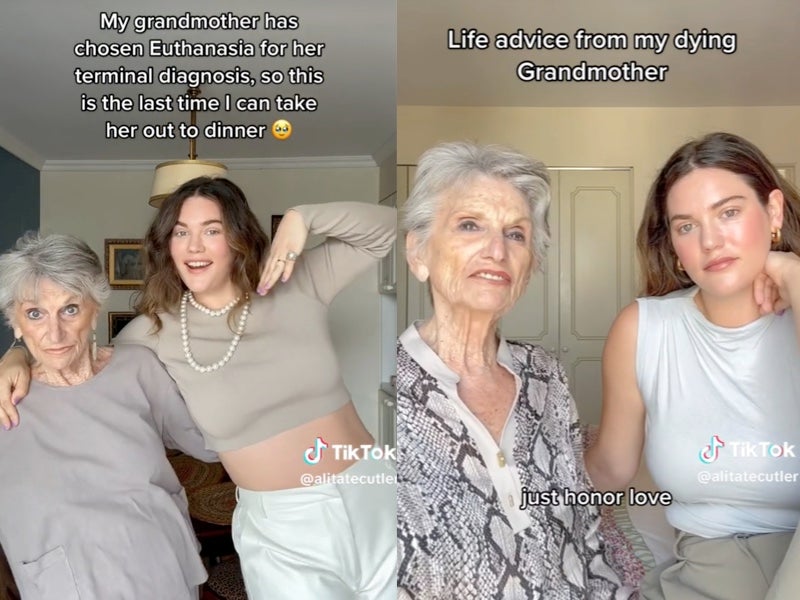The image consists of two TikTok screenshots featuring a touching moment between a grandmother and her granddaughter. In the left image, the title reads, "My grandmother has chosen euthanasia for her terminal diagnosis, so this is the last time I can take her out to dinner," accompanied by a crying emoji. The scene shows an elderly woman with gray hair, wearing a gray top, looking into the camera. Beside her is her granddaughter, a younger woman with long brown hair, dressed in a gray top, white pants, and a white pearl necklace with round beads, lovingly holding her grandmother's shoulder. They are in a house setting with white walls adorned with paintings.

The right image, titled "Life advice from my dying grandmother," reflects a poignant message, "Just honor love." Here, the same elderly woman is seen wearing a black and white patterned shirt, and beside her stands her granddaughter, now wearing a white top and gray pants. The granddaughter's expression has shifted to a more pensive look. The TikTok username, "Alita A. L. Cutler," is displayed, framing their shared moment of love and reflection.